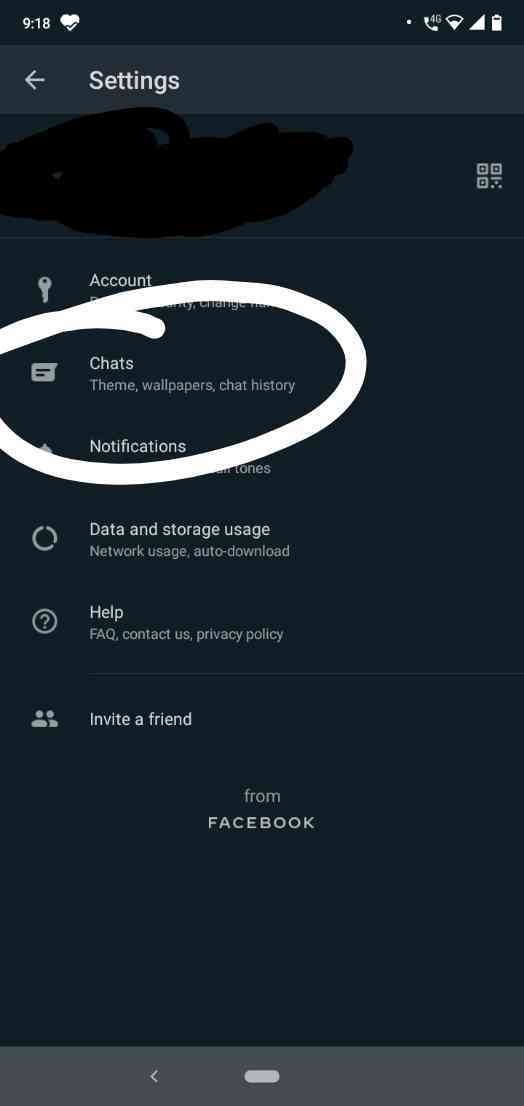The image displays a smartphone screen featuring a settings page, likely from the Facebook application. The background is dark blue, providing a stark contrast to the white text and icons. At the top left of the screen, the time is shown as 19:18, accompanied by a heart icon. On the top right corner, there are indicators for a 4G call, WiFi connection, and network strength, along with a bird icon.

Beneath the header, the settings menu is displayed with various options including "Account," "Chat," "Notifications," "Data and Storage Usage," "Help," and "Invite Friend," all written in white text. A prominent white circle is drawn around the "Chat" and "Notifications" options, highlighting these specific settings. The details beneath these options are slightly obscured due to the circle, which seems to focus the viewer's attention on these sections.

Under "Chat," there are further options labeled "Theme," "Wallpapers," and "Chat History." The "Data and Storage Usage" section includes sub-options like "Network Usage" and "Downloads." The "Help" section lists "FAQs," "Contact Us," and "Privacy Policy." At the very bottom of the menu, the option "Invite Friend" is visible, followed by a small note that reads, "From Facebook." 

Overall, this detailed image effectively captures the layout and specific settings available within the Facebook application's settings menu on a smartphone.